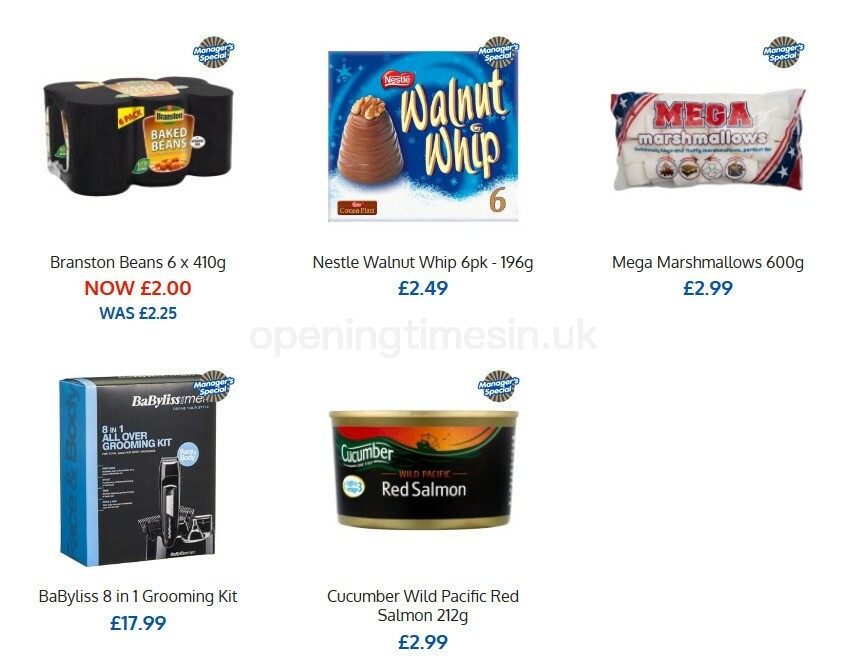This webpage displays various food items along with one grooming kit, all marked with "Manager Special" discounts. A watermark reading "openingtimesyn.uk" sits prominently in the middle of the screen.

In the first row, three items are showcased:
1. **Baked Beans:** A six-pack of Branston Baked Beans, each can weighing 410 grams. The packaging is black with the label "Baked Beans" and priced at £2.00 from an original £2.25.
2. **Walnut Whip:** A Nestlé Walnut Whip six-pack, totaling 196 grams. The item is marked at £2.49.
3. **Mega Marshmallows:** A 600-gram pack of Mega Marshmallows priced at £2.99.

In the second row, two items are presented:
4. **Grooming Kit:** The BaByliss for Men 8-in-1 Grooming Kit, priced at £17.99.
5. **Red Salmon:** Cucumber Wild Pacific Red Salmon, weighing 212 grams and priced at £2.99.

Each item prominently displays the "Manager Special" icon, indicating special pricing.